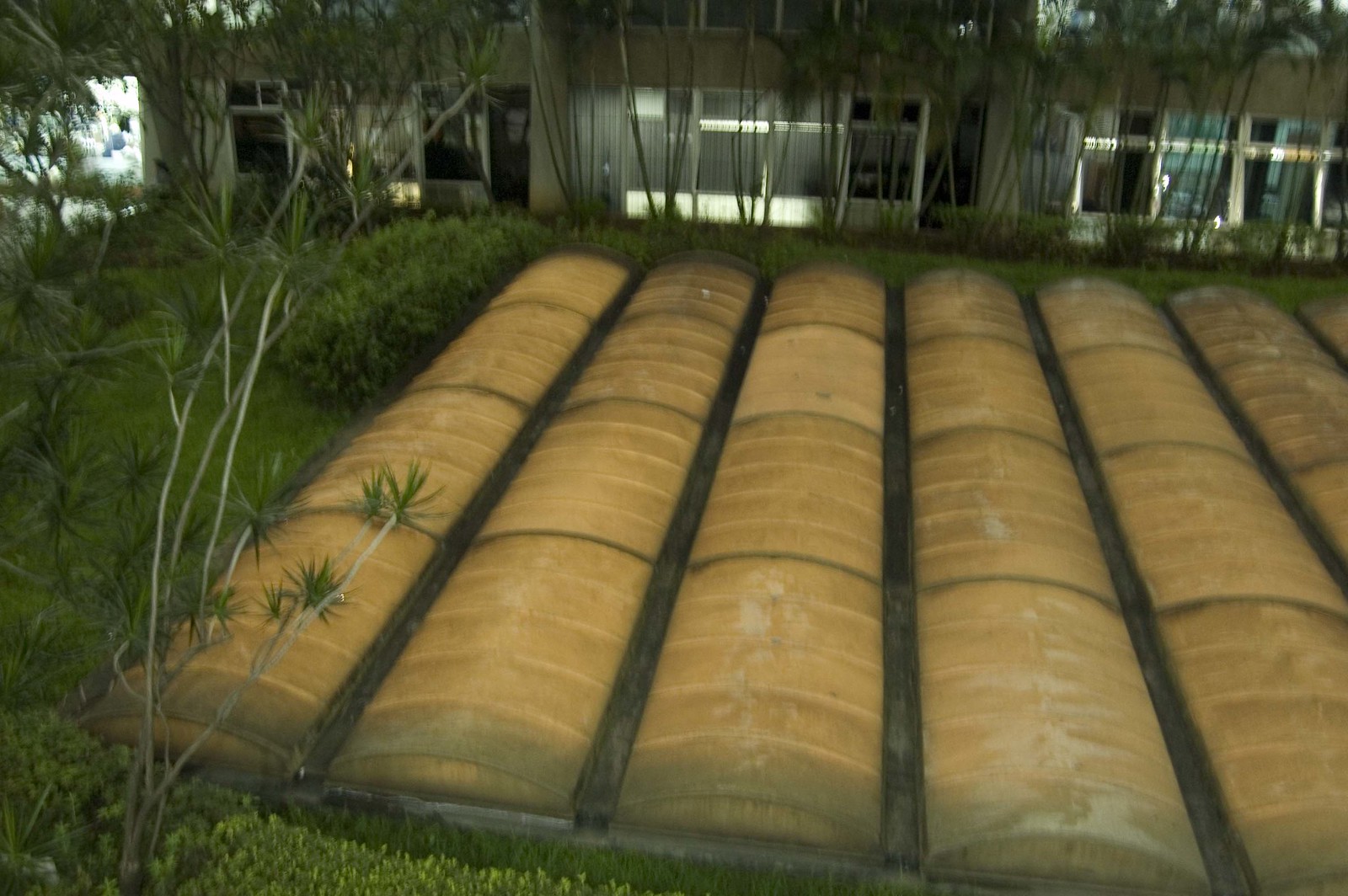The image captures an exterior scene believed to be situated outside an office or residential complex. Despite the slightly unfocused quality, the vivid lush greenery is evident with abundant grass, bushes, and thin trees populating the space. The foreground presents rows of unusual structures that resemble arched, brownish-tan panels, each lined with metal separators. These panels, possibly solar or crop covers, extend approximately 24 feet long and 2.5 feet wide, totaling around 20 to 30 in number. Behind these structures, multiple building facades, likely office fronts, are visible, framed by a line of trees. Additionally, to the left of the image, a large raspberry bush suggests that the area may support subtropical vegetation.